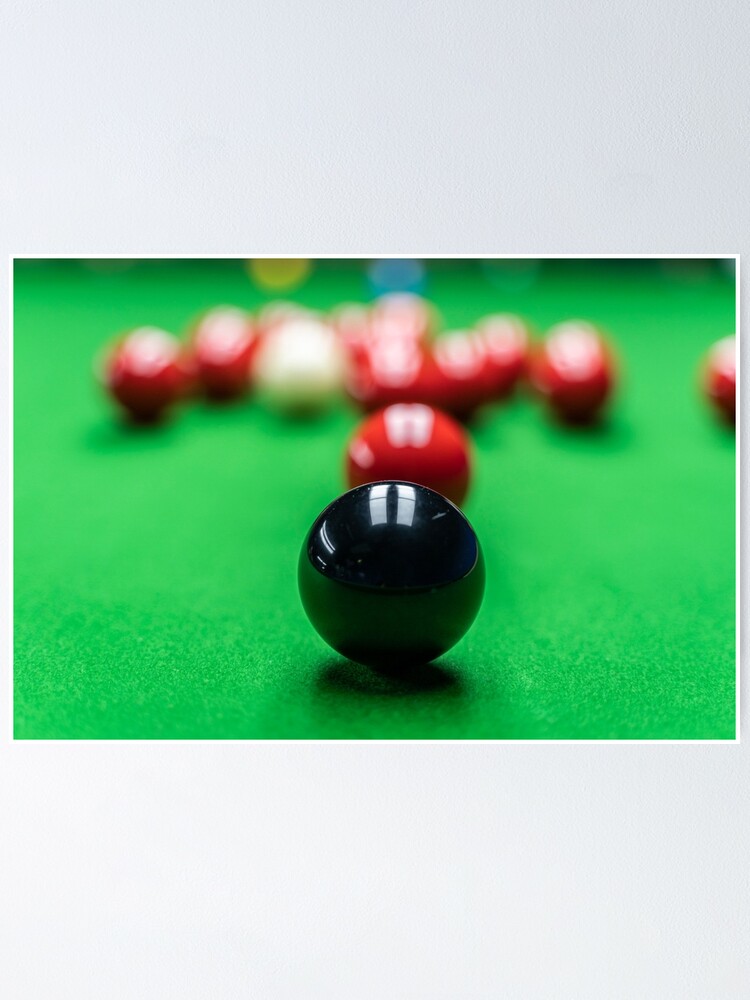The image features a green snooker table set against a grey background, with a prominent white outline framing the central photograph. The focal point of the image is a glossy black snooker ball situated near the bottom center, capturing light reflections. Directly behind the black ball is a red ball, followed by a nearly straight line of additional red balls extending further into the background. To the left of the black ball is a white cue ball, and slight blue and yellow distorted circles can be seen behind the red balls. The green felt surface of the table contrasts sharply with the vividly colored balls, creating a striking visual composition. The edges of the image show blurred portions of red and other colored balls, adding depth and focus to the central elements.